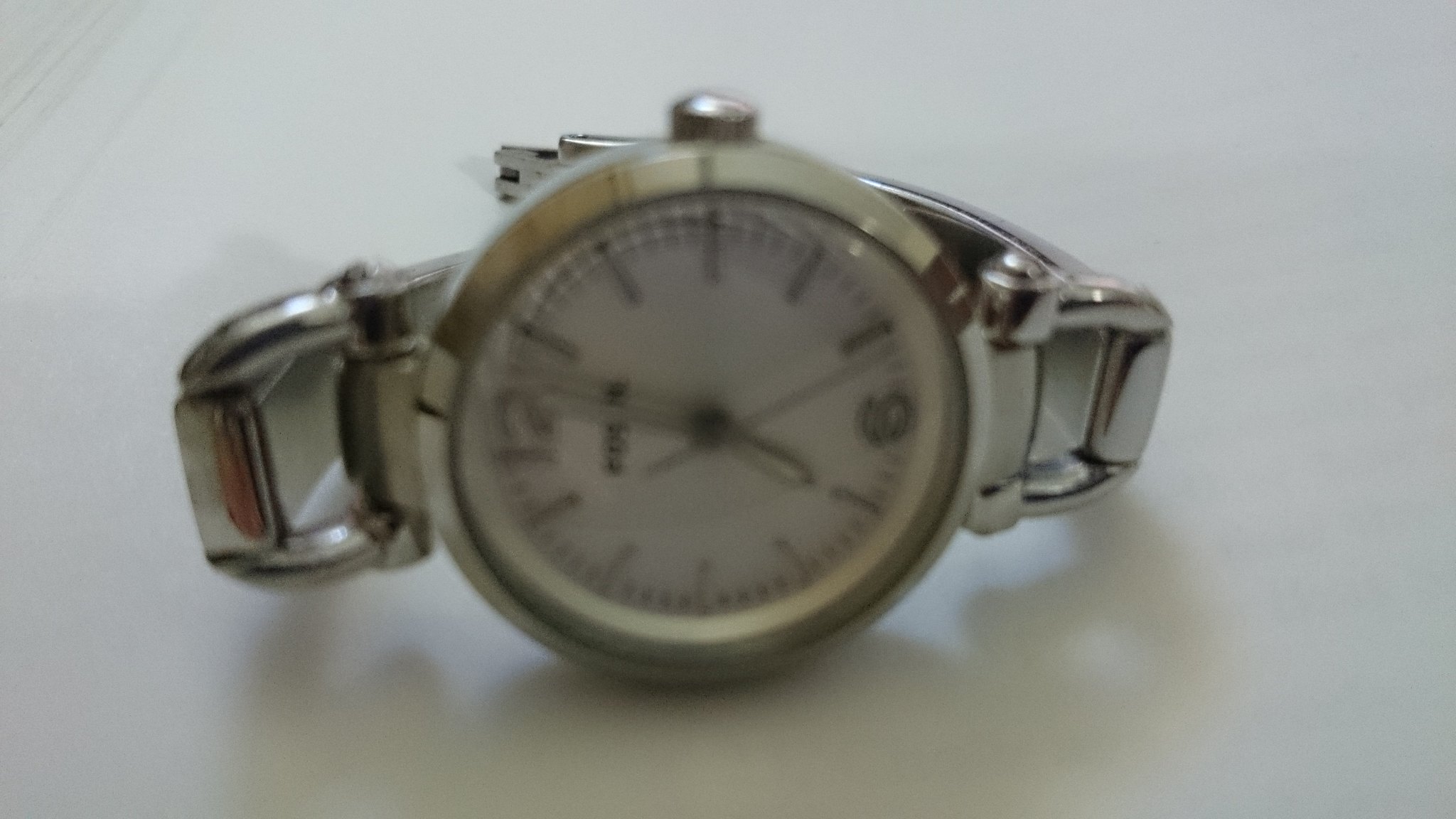This photograph features a close-up of a silver-colored metal wristwatch, positioned centrally on a white, marbled tabletop. The watch, which is not being worn and casts a faint shadow on the table, has a reflective, shiny, and chrome-like appearance. The circular bezel around the face, the time-adjusting knob, and the band are all made of the same silver metal.

Despite the overall blurriness of the image, certain details are discernible. The watch face is white, with fine lines marking the minutes and hours. There are no visible numbers except for the 12 and 6, which are faint due to the haziness. Additionally, some text near the 12 is present but indistinguishable. The watch features all three hands: the hour, minute, and second hands, each pointing in different directions. The face of the watch also exhibits a slight yellow tint. Notably, there is a significant gap visible near the hinges on both the left and right sides of the watch.